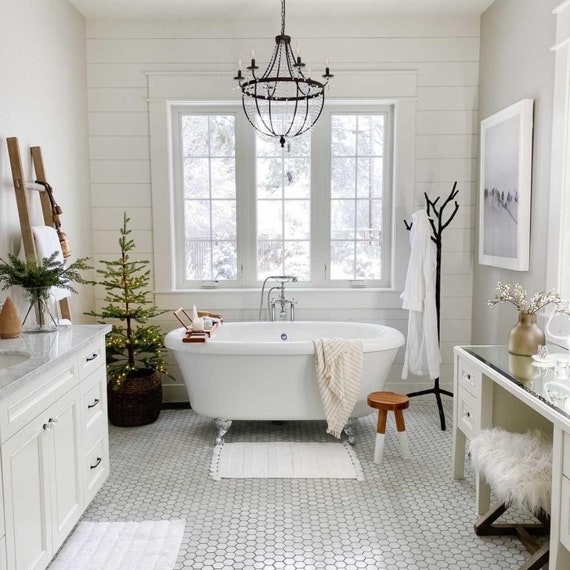This photograph captures the serene interior of a rustic yet elegant bathroom. The centerpiece is a medium-sized, white bathtub positioned under a large window with three panes, offering a glimpse of a picturesque winter wonderland outside. The bathtub, accentuated by chrome feet and a silver faucet, is complemented by a distinctive black chandelier hanging overhead. A feature of the bathroom is a unique black tree-shaped rack, located in the right fore corner, adorned with a white bathrobe. Nearby stands a small, festive fake pine tree, adding a seasonal touch.

The bathroom’s flooring consists of a classic white hexagonal tile pattern, and the walls are predominantly white with the fore wall distinguished by wood shingles. The ceiling shares the uniform white color of the surrounding walls. A notable grey marble countertop adorns the sink on the left, paired with white cabinets, while a makeup vanity with a furry stool resides on the right. Completing the decor, a painting is hung on the left wall. The cohesive blend of textures and elements creates a refined yet cozy ambiance.